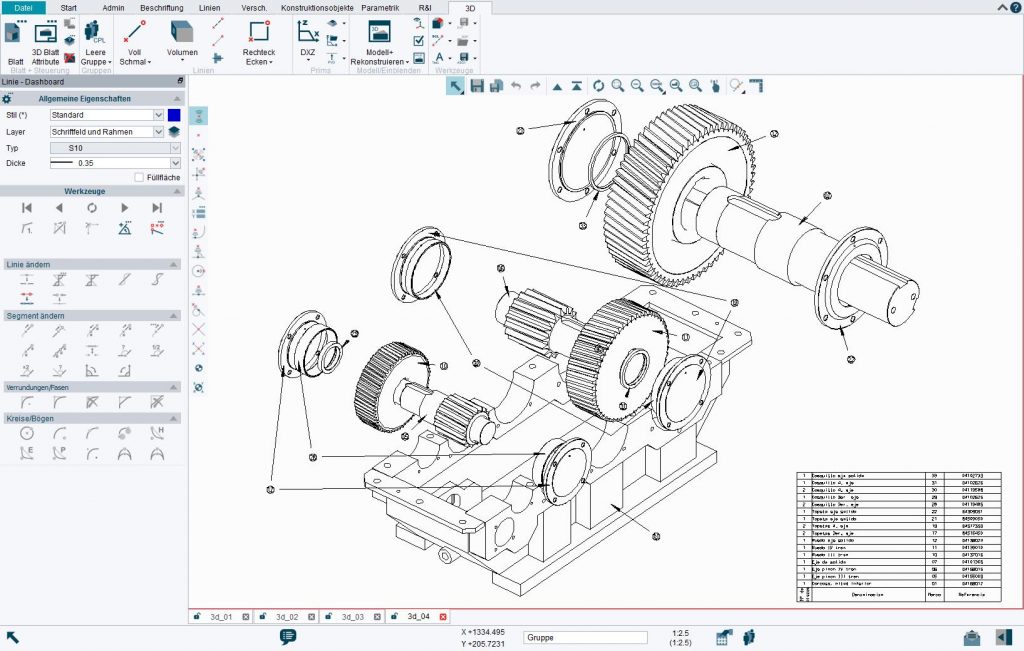The image is a computer screenshot displaying a detailed diagram of a mechanical device, featuring several gears, cogs, and various circular washers. The screenshot seems to be taken from a 3D design program, possibly in a foreign language such as German. The interface resembles design software like WordPerfect or similar. The diagram shows how different parts fit together with numbers labeling each component. The top and left sides of the screen contain various controls and editing tools, suggesting that the user can modify the design. At the bottom right, there is a chart or key that lists and explains the numbered parts of the machinery. The diagram is mainly in black and white, with multiple arrows pointing to specific components, illustrating their interconnections and functions.